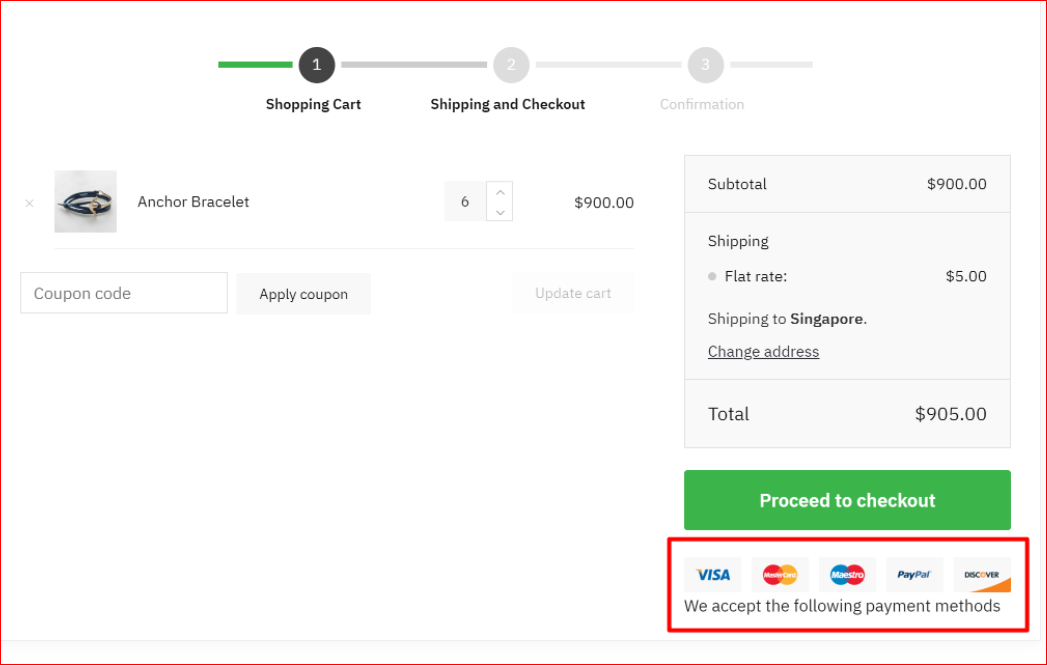A meticulously edited screenshot captures the checkout section of a jewelry store's desktop website, set against a sleek white background. Dominating the image are two prominent red boxes, digitally highlighted for emphasis. The largest outlines the entire checkout box, while the second frames the payment method section positioned at the bottom right. Here, logos for Visa, MasterCard, PayPal, and Discover are displayed beneath a bold, gray inscription reading "We accept the following payment methods."

Central to the image's upper portion, three black circles with ascending white numerals (1, 2, and 3) delineate the checkout steps. A horizontal line connects these circles, transitioning from green at the leftmost end by the numeral 1 to a continued progression rightward. The number 1 circle is distinct in bold black, while the 2 and 3 circles remain grayed out, indicating progressive steps.

Beneath this navigational guide, the left side features a small thumbnail of an anchor bracelet, adjacent to the item's description. Next to it, a box displays the quantity '6,' flanked by up and down arrows allowing for adjustment. To the right, the price is marked as $900 in prominent black digits. Below, an input field labeled "coupon code" sits beside a clickable "apply coupon" button. 

Further right, a summary box details the cost breakdown: "Subtotal $900," "Shipping: Flat rate $5 (shipping to Singapore)," accompanied by a "change address" option. At the bottom left, 'Total' is stated, counterbalanced on the right by the total cost of $905. A large green "proceed to checkout" button concludes the interface at the bottom, inviting the final step in the purchasing process.